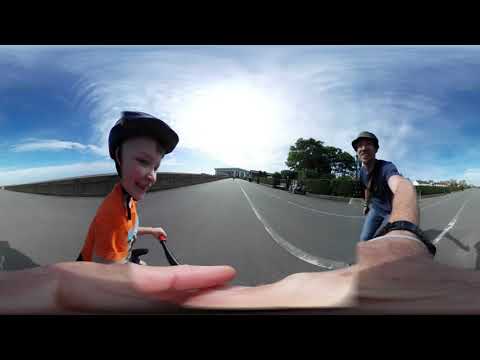The panoramic photograph shows a man and a young boy, possibly his son, standing on a winding road on a clear, sunny day. The top and bottom of the image are bordered by thin black rectangles, creating a wide, rectangular frame. The bright blue sky dominates the top half of the image, with a particularly white, radiant area in the center. The road occupies the bottom half, curving from the left to the horizon and then to the right, marked by white lines. The boy appears slightly distorted on the left side of the image, standing on a bicycle with a black helmet and wearing an orange shirt with a graphic in blue and black on the chest. The man stands to the right, dressed in a green hat, a navy blue short-sleeve shirt, blue jeans, and a black watch on the wrist of the hand holding the selfie stick, possibly capturing this moment. The background includes trees, business-like buildings, and distant hills, adding depth to the scene.